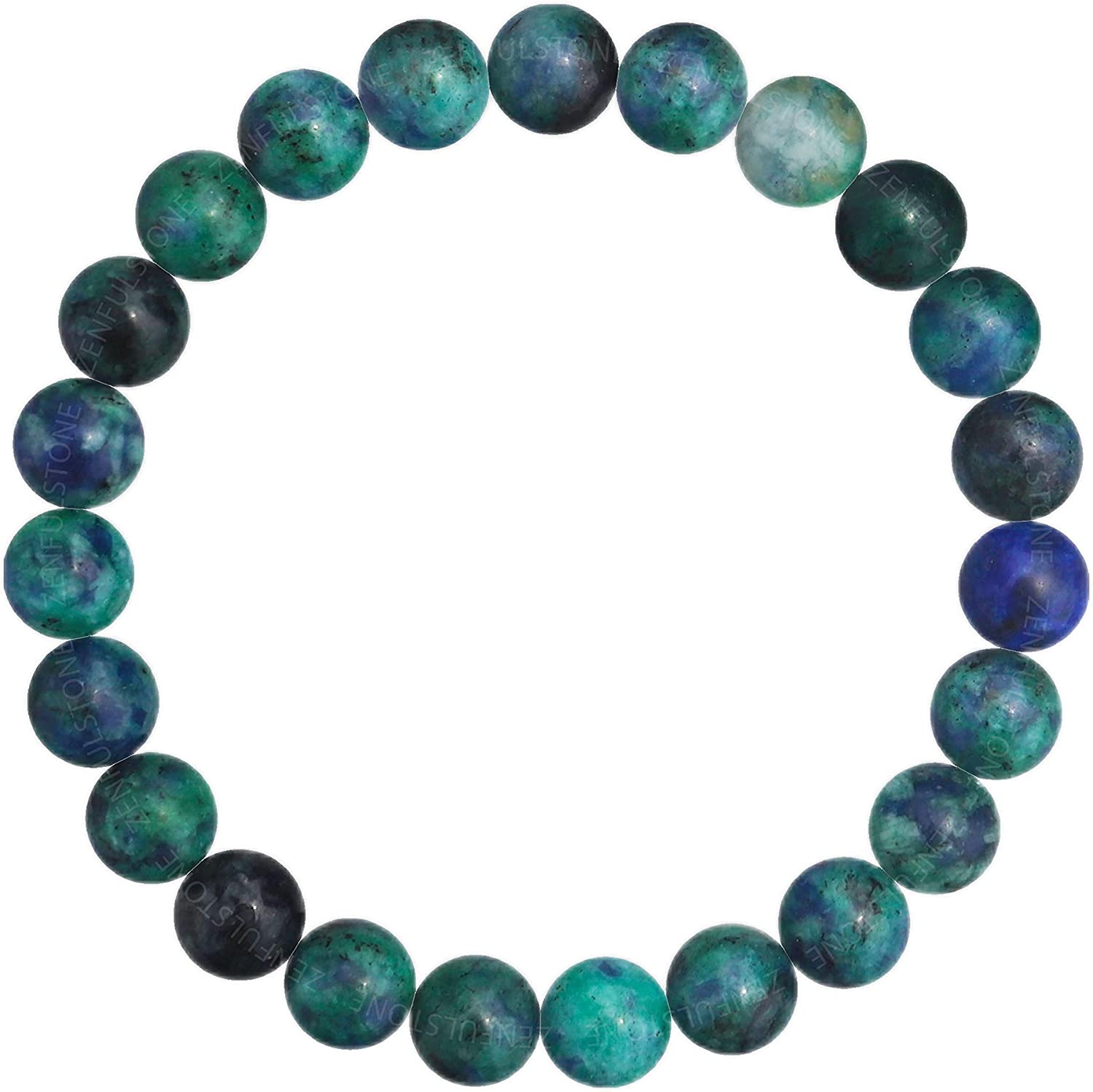This image features a piece of jewelry, likely a beaded bracelet, set against a plain white background. It is composed of 22 interlocking beads forming a complete circle. The beads vary in shades of blue and green, with a stronger tendency towards blue. Some beads are dark and opaque, while others are translucent, giving a potential glimpse through them. Each bead is unique in color and appearance, with a shiny texture suggesting they might be made of glass, plastic, or stone. The beads' appearance is reminiscent of tiny planets viewed from space. The material connecting the beads is not visible, but it is implied to be an inner string or rubber band.